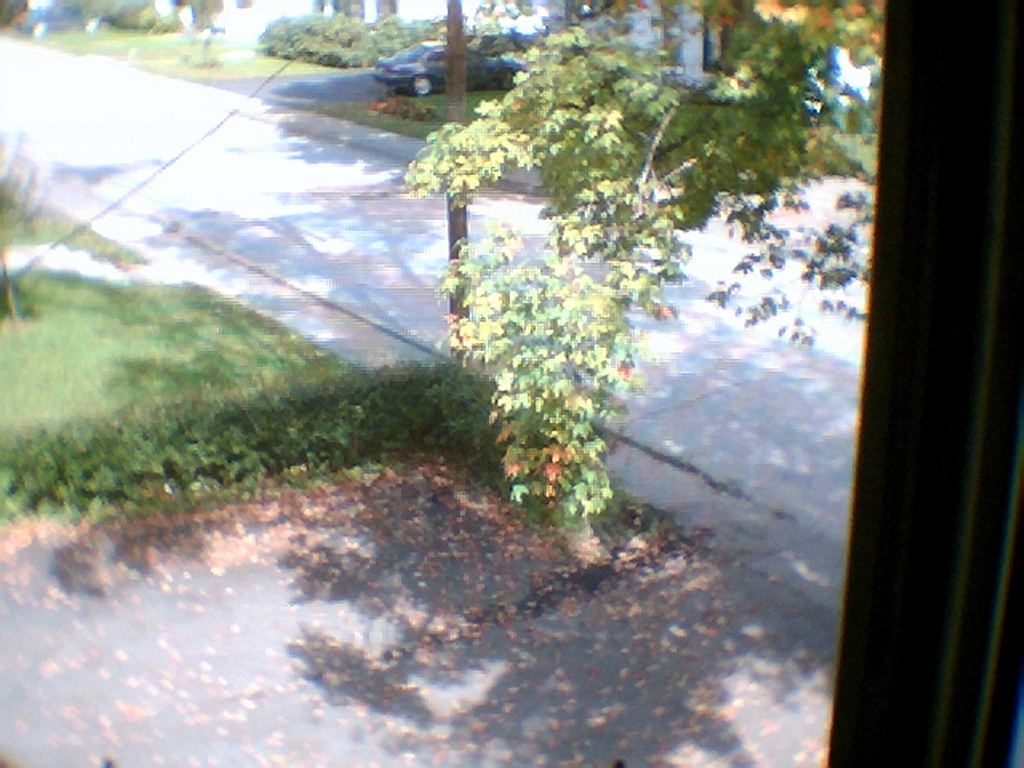This is a blurry photograph that appears to have been taken through a house window, creating an almost watercolor-like effect as if it might have been put through a filter. The image, reminiscent of an early 2000s camera phone picture, shows an autumn scene outside. The window frame is brown, partially visible on the right-hand side. Through the window, you can see a driveway covered in fallen leaves, leading to a small residential street. The driveway, made of light gray asphalt, opens onto a narrow street with a layer of grayish asphalt. 

On one side of the driveway is an L-shaped green hedge, and beyond that, a green lawn stretches out with scattered foliage. A sidewalk runs between the lawn and the street. Shadows are cast by the large tree in the foreground, whose branches and leaves, a mix of green, orange, and red, hang over the driveway. In addition, a skinny brown telephone pole and telephone wire are visible, indicating a residential area. Across the street, there is a White House and several vehicles, including a grayish car parked in what appears to be a small parking lot. The overall scene is suggestive of a typical New England neighborhood on a sunny fall day.